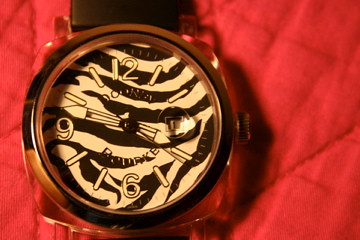The image showcases an elegant watch resting on a vibrant red fabric. The fabric, possibly a blanket, features distinctive stitching in a triangular pattern, adding texture to the scene. Only a section of the fabric is visible, leaving its full identity ambiguous. The watch itself is adorned with a black band peeking out from the top of the frame. The timepiece has a striking square-shaped outer case in gold, complemented by a matching gold turn-dial on the side. Encircling the inner face is a gold rim, framing a unique zebra print dial. The dial prominently displays the numbers 6, 9, and 12, with subtle off-white hash marks indicating the remaining hours. The watch hands are also off-white, blending slightly with the dial's pattern, which makes it somewhat difficult to read the time at a glance.